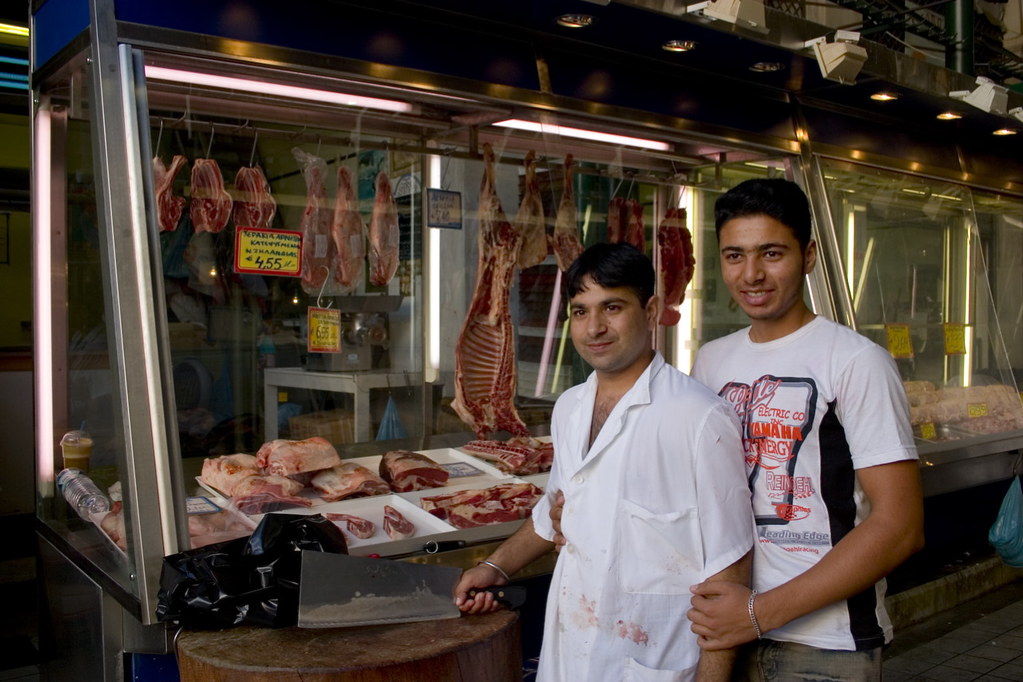The photograph captures two men, possibly in their late 20s or early 30s, standing closely together in what appears to be a bustling marketplace, specifically a butcher shop. 

The man in front is wearing a white button-down collared shirt that looks slightly flowy. He has dark hair and holds a large butcher knife in his right hand; his shirt appears to have splashes of blood on it, suggestive of his role as a butcher. The lighting enhances the scene, with glass-fronted refrigerated cabinets filled with chunks of meat visible around them.

Standing closely behind, another man with dark hair is dressed in a white t-shirt adorned with an orange, black, and white graphic logo. He is medium-skinned and smiling at the camera, while both his left hand and his right arm gently hold the man in front. The background features additional meat hanging and trays of prepared cuts, further emphasizing the butchery setting. Both men's smiles suggest camaraderie amidst their busy work environment.